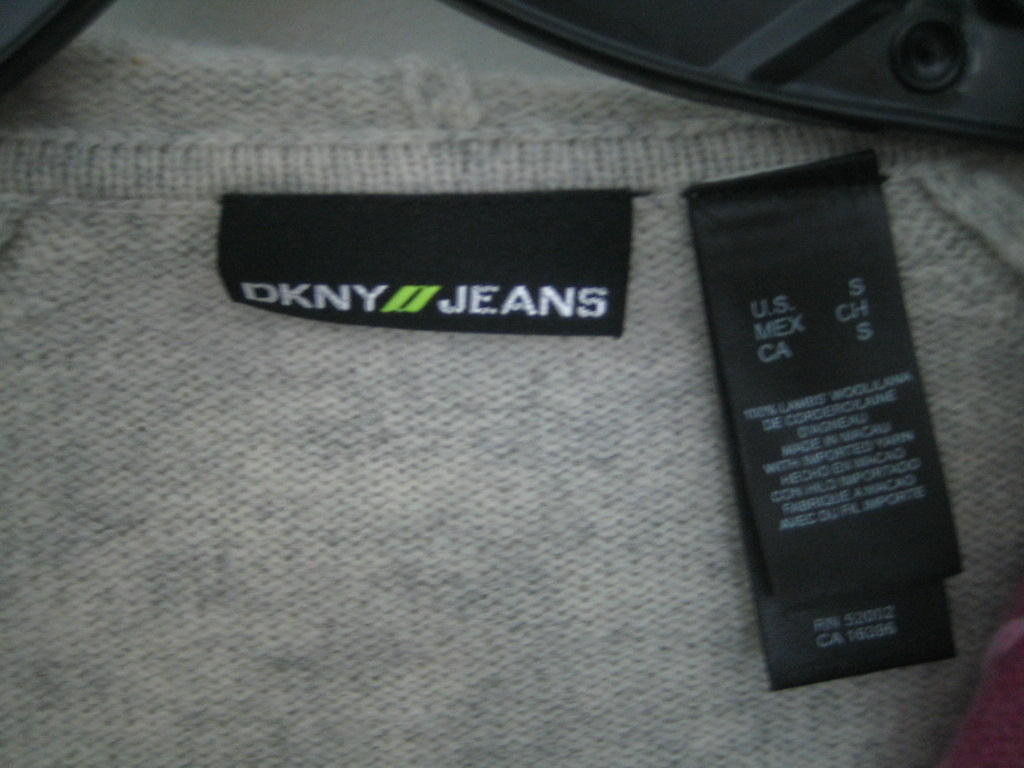A detailed close-up image of clothing tags attached to a gray sweatshirt.  The photo centers on the collar area, where a black tag with white text 'DKNY JEANS' prominently stands out. Between the words 'DKNY' and 'JEANS', there is a green, slanted line symbol. To the right of the brand tag, another label is visible, which appears to contain washing instructions. The image also shows fragments of a plastic hanger, with parts coming into view at the top, top-right, and top-left edges of the frame, hinting that the sweatshirt is hung up.